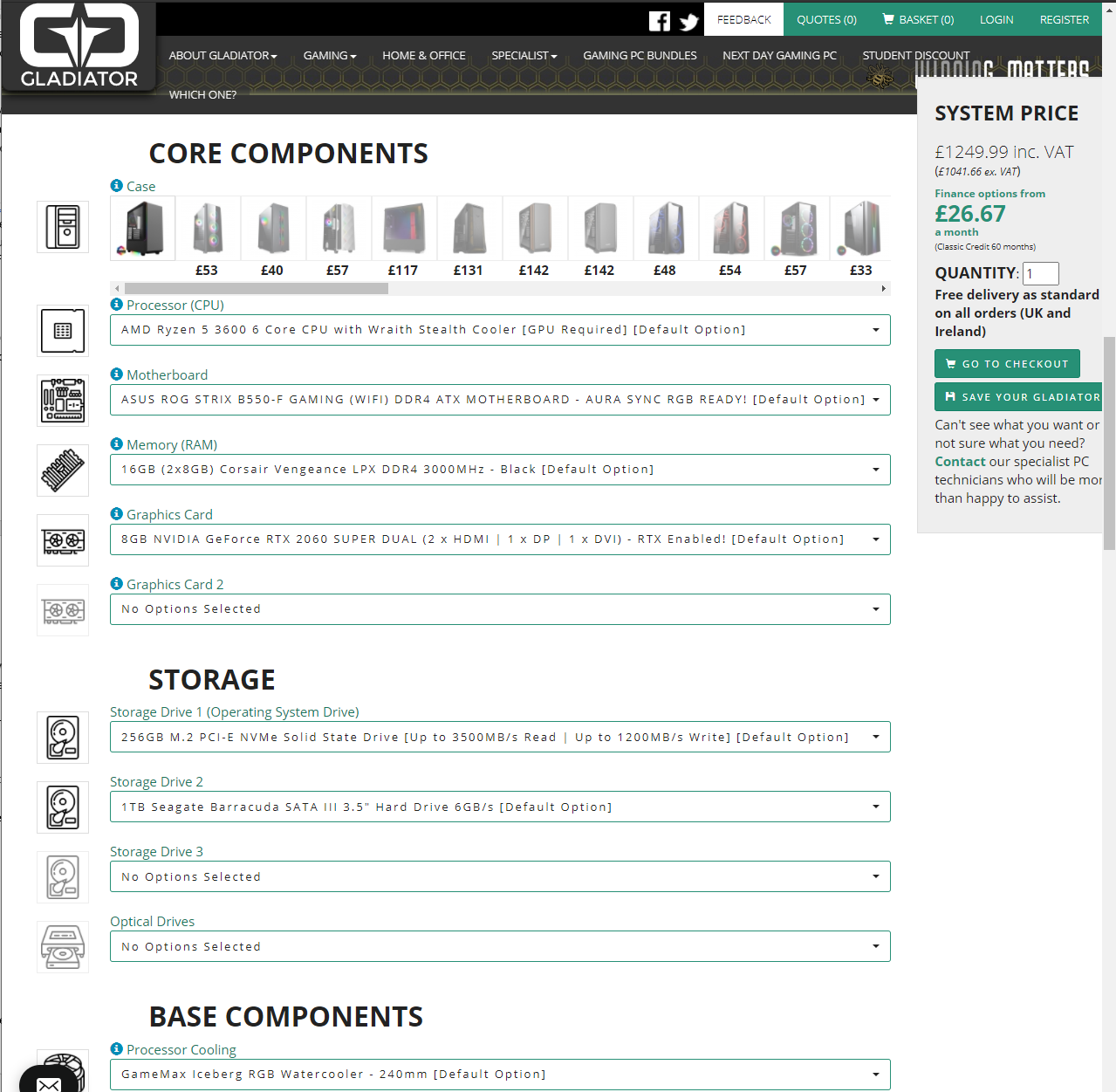This image is a detailed screenshot of a website named Gladiator, presumably an e-commerce platform specializing in computer components. At the top, a sleek logo features a minimalist white illustration and the name "Gladiator," all set against a grey background. Adjacent to the logo are black-and-white icons for Facebook and Twitter, indicating social media integration.

The navigation bar includes options such as "Feedback" displayed in black ink on a white background, and "Codes," "Baskets," "Register," and "Login," all written in white ink against a green background. This layout suggests user-friendly access to various site functions.

The primary content of the site appears to focus on selling essential computer components, as evidenced by sections labeled "Core Components” in black ink. These sections list different product types and prices, organized under categories such as "Storage" and "Base Components." A floating pop-up displays a system price, offering a snapshot of current deals or selections.

Most textual elements are rendered in grey ink, with some highlighted in black for emphasis. Prices are marked in green ink, and important actions such as "Go to Checkout" and "Save Your Gladiator" are set against green backgrounds, ensuring they stand out for ease of navigation. This comprehensive layout indicates a dedicated platform for purchasing computer hardware.